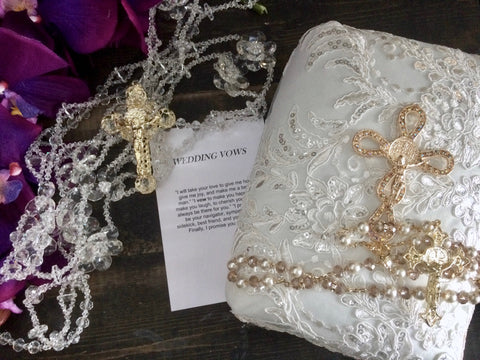In the image, there is a piece of paper at the center titled "Wedding Vows," featuring eight lines of small, unreadable black text likely containing the vows. To the right of the vows, there is a white package adorned with intricate floral and leafy decorations. Below the package lies a necklace featuring a cross made of white and yellow beads or pearls. On the left side of the wedding vows, there's another golden cross decorated with small gems, attached to a long string of what appear to be diamonds. Further to the left, a cluster of large, vibrant purple leaves or shapes is resting on the surface of the table, creating a striking contrast with the other items in the scene.